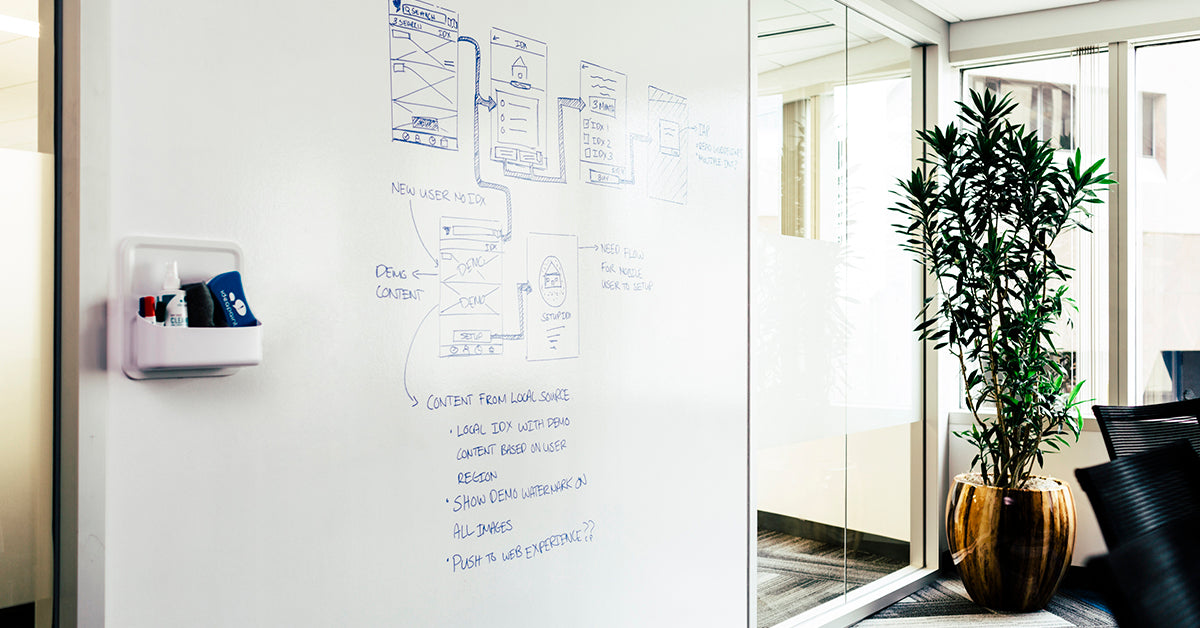The image depicts an indoor office space bathed in daylight, likely taken during the day. The scene is dominated on the left side by a floor-to-ceiling whiteboard filled with detailed mechanical drawings and annotations in blue ink. Specific noted text includes "content from local source local IOX," and phrases related to user interaction and demo content. The whiteboard features a small holder for markers and erasers on its far-right edge. On the right side of the image, a large, green bamboo-style plant is housed in a bronze vase, positioned near a window that offers a view of adjacent building windows. Adjacent to the plant are three black chairs positioned on a black-and-white carpet. The scene also includes a mirror, adding to the depth and brightness of the room.